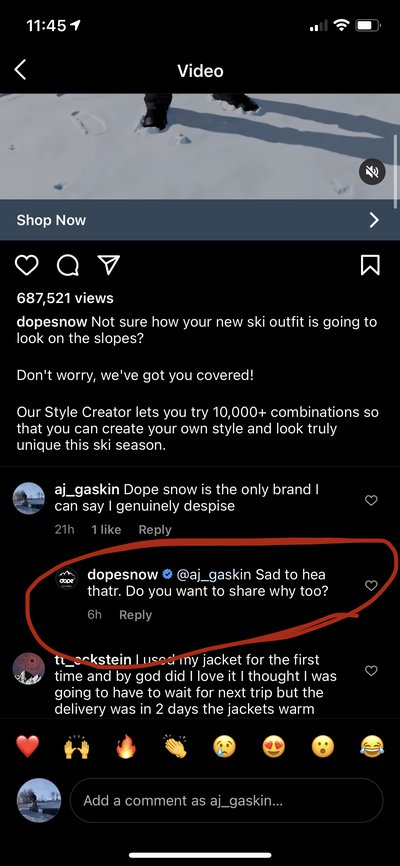**Caption:**

The image captures a screenshot of an Instagram post viewed on a mobile phone with a dark theme enabled. The phone’s user interface displays a white header with the time set at 11:45 AM on the left, accompanied by a location icon. On the top right, the signal strength shows 2 out of 4 bars, the Wi-Fi icon indicates an active connection, and the battery icon indicates approximately 70-80% charge.

Just below the header, the screen shows the Instagram navigation bar with a white arrow pointing left and the word "Video" centered. The main focus of the screenshot features the lower part of an Instagram image post, showcasing a pair of sneakers standing in freshly fallen snow, with visible footprints. A "Shop Now" button is displayed prominently at the bottom of the image.

Directly beneath the image, Instagram's reaction bar appears in white, featuring the heart icon (for likes), the comment icon, the forward icon, and the bookmark icon. The post boasts an impressive 687,521 views.

The description provided by "Dopesnow" reads: "Not sure how your new ski outfit is going to look on the slopes? Don’t worry, we’ve got you covered. Our style creator lets you try 10,000+ combinations so that you can create your own style and look truly unique this ski season." This is followed by the comments section.

Highlighted in the comments is a remark by AJ Gaskin stating, "Dope snow is the only brand I can say I genuinely despise." The official and verified account of Dope Snow replies, "Sad to HEATHATR. Do you want to share Y2?" (Note: The reply includes a typo likely meant to read, "Sad to hear that. Do you want to share why?")

The screenshot prominently circles the replied comment to draw attention to Dope Snow's response. Below the comments section, the screenshot shows the option to add a comment, indicating the user as AJ_Gaskin, who is the same person that made the original comment and captured the screenshot.